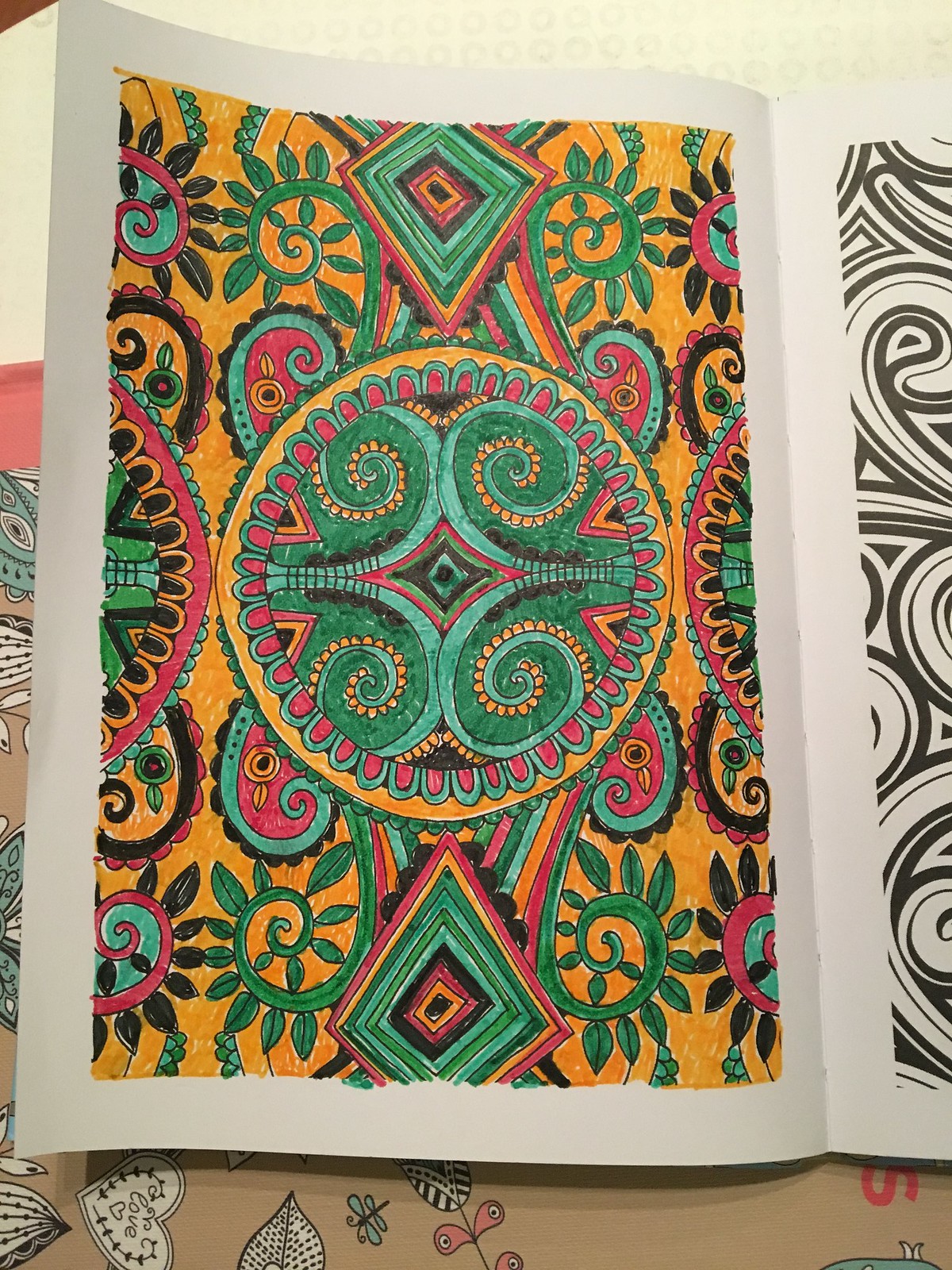In this image, we see an open coloring book showcasing intricate artwork with geometrical and floral designs. The left page is partially colored, displaying vibrant hues of green, red, yellow, and black that bring to life round circular medallions and intertwining vines, creating a captivating and colorful scene. The right page is visible only in part and remains uncolored, offering a contrast to the completed artwork. The coloring book rests on a background of brown wrapping paper, adorned with small, charming illustrations of hearts, bugs, and flowers. These whimsical details peek out from the edges of the coloring book, adding an extra layer of interest to the photograph.